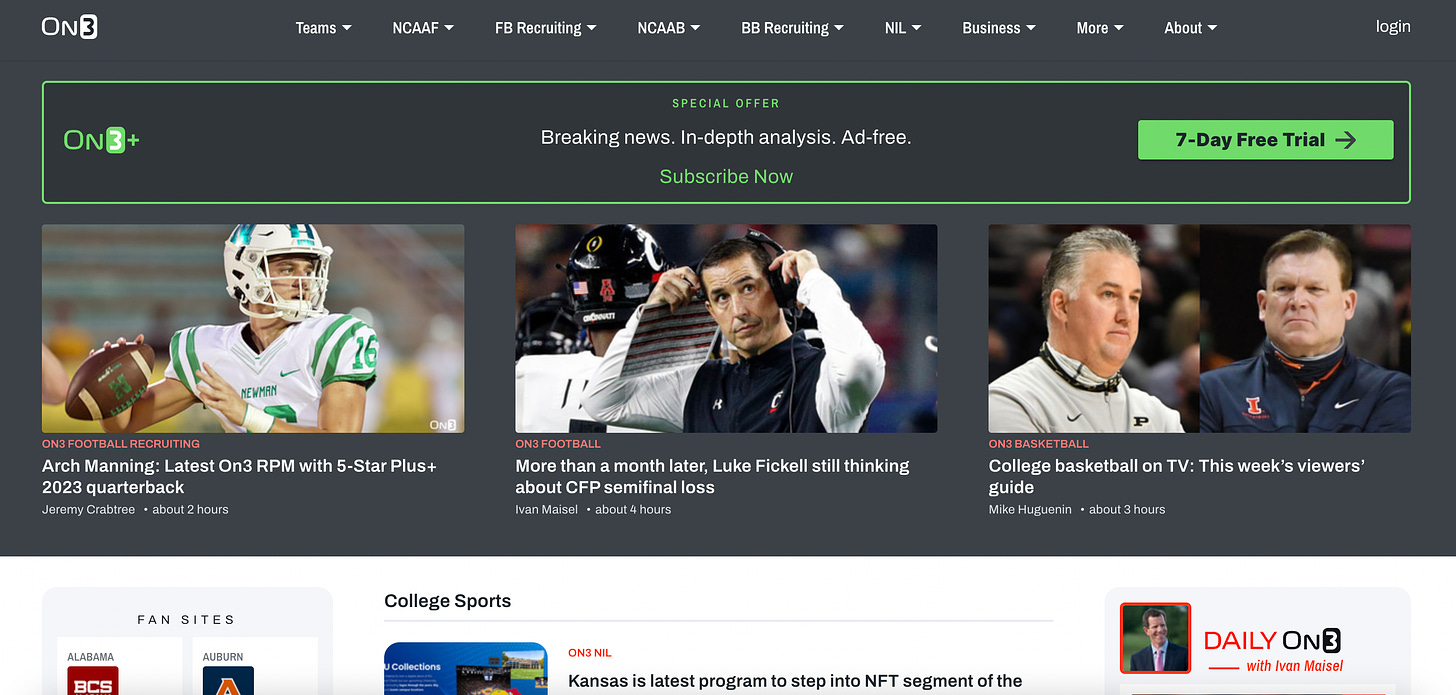The image is a detailed screenshot in landscape mode comprising two main sections. The larger upper section features a dark green background while the smaller bottom section stretches across from the bottom left to the bottom right.

In the bottom section, starting from the left, there's a white background area containing a small gray card. This card is divided into two parts: "Fan Sites" on the left, and "Alabama" and "Auburn" on the right. Moving right, another labeled section reads "College Sports," though it is partially cut off and would continue down if the page were scrolled. Below this, there's a headline stating "ON3NIL: Kansas's latest program to step into NFT segment." On the far right, the phrase "Daily ON3 with Ivan Maisel" is visible.

The main section, occupying the top part of the screenshot, begins with the "ON3" logo in the upper left corner. Adjacent to it are several category headings with dropdown arrows: "Teams," "NCAAF," "FB Recruiting," "NCAAB," "BB Recruiting," "NIL," "Business," "More," and "About." The upper right-hand corner contains a "Login" button.

Directly below, a light green bar spans the entire width, highlighting special subscription offers. The text within the bar reads:
- In green, "Special Offer."
- In white, "Breaking News, In-Depth Analysis, Ad-Free."
- Back in green, "Subscribe Now" (on the right side). 
Within this green rectangle, there's a green button featuring large letters stating "7-day free trial" alongside a right arrow.

Underneath, three thumbnails appear, likely linking to videos. The titles for these videos are:
1. "Arch Manning, Latest ONR PM"
2. "More than a Month Later, Luke Fickle"
3. "College Basketball on TV"

Overall, this organized and visually segmented layout provides quick access to various categories, headlines, and subscription offers, enriched with multimedia content.